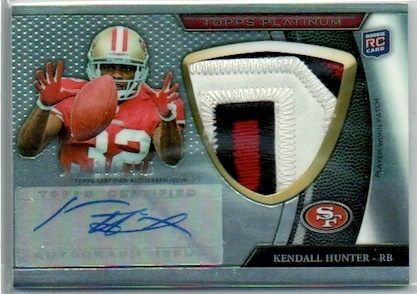This image is that of a horizontally oriented Topps Platinum football card, encased in a clear plastic sleeve. Dominating the left side of this card is an action shot of football player Kendall Hunter, a black male donning a red jersey emblazoned with the white number 32. Hunter, a player for the San Francisco 49ers, is depicted with his hands outstretched and fingers spread wide, poised to catch a football flying towards him. He sports a golden helmet with a red and white stripe down the center and wears red gloves to match his vibrant jersey. Below the dynamic image, there's a signature in blue pen, signifying its collectible value.

On the right side of the card, there's a gold-colored crest featuring a small window showcasing a patch of fabric from Hunter's actual game-worn jersey, with visible stitching of the number zero from the jersey. Adjacent to this patch, in small vertical black lettering, it reads "Player Worn Patch." The card also includes the San Francisco 49ers' traditional logo set inside a circle and, within a black bar at the bottom right, the text "Kendall Hunter - RB" (denoting his position as running back). At the top of the card, set against a burgundy background with gold text, is the title "Topps Platinum" signifying the premium quality of the card.

Overall, this card meticulously blends aesthetic elements and collectible features, epitomizing sought-after sports memorabilia.